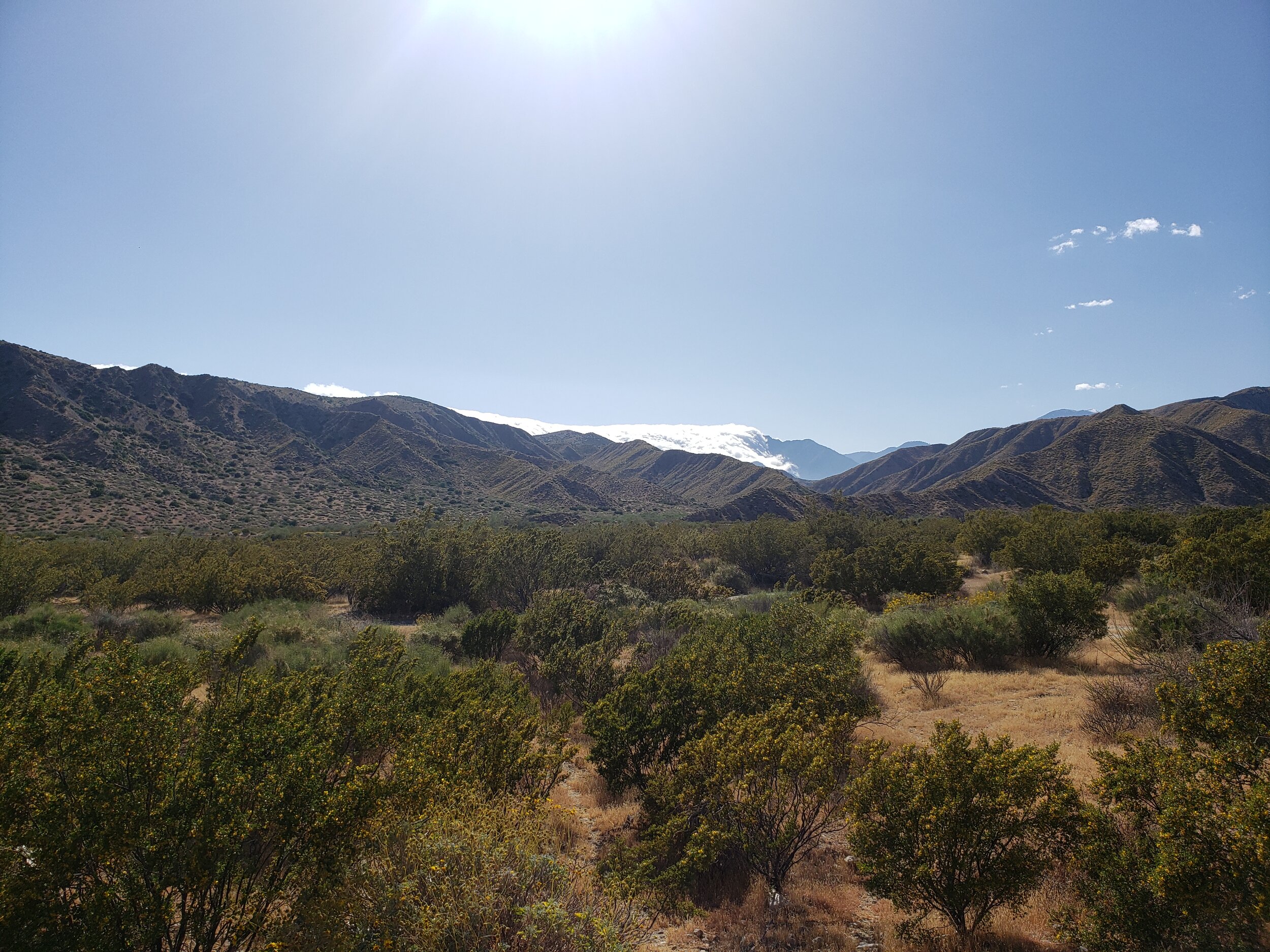The image depicts a vast desert landscape characterized by a clear blue sky with a few wispy clouds on the right-hand side. The sun, partially visible at the top, casts its rays downwards, suggesting it's midday. Dominating the foreground is a brown desert floor interspersed with patches of dead-looking grass and green shrubs adorned with small yellow blossoms. On the left side, more green shrubs and some weathered trees rise from the rugged, jagged hills. These hills transition into a series of low, brownish mountains. In the background, a snow-capped mountain range looms, adding contrast with its wide, white-topped peaks. As the terrain extends further back, more mountains appear as distant shadows, creating a layered effect. The general impression is one of stark beauty, combining the harshness of the desert with the serene presence of the mountainous backdrop.